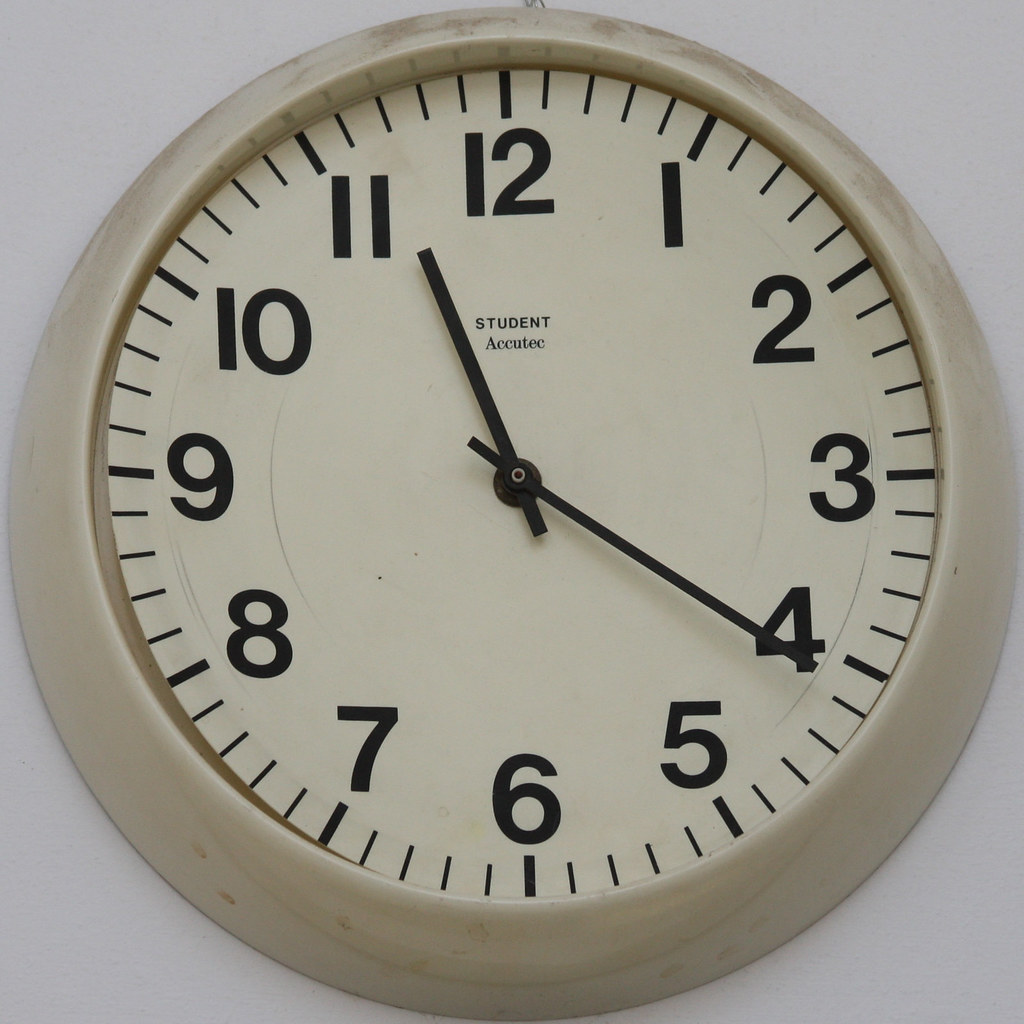This photograph features a prominently displayed circular wall clock against a smooth, white wooden wall. Dominating about 90% of the image, the clock’s outer border is a slightly dirty off-white or tan color with brown markings. The lighter off-white interior forms a contrast to the surrounding frame. Bold black numbers from 1 to 12 are evenly spaced around the clock face. The shorthand is positioned slightly past the 11, and the longhand rests just after the 4, indicating the time is 4:57 PM. Notably, under the number 12, the clock face reads "student Acutech" in small, black text. The four corners of the image reveal the light gray backdrop of the wall, emphasizing the clock's circular shape and detailing.